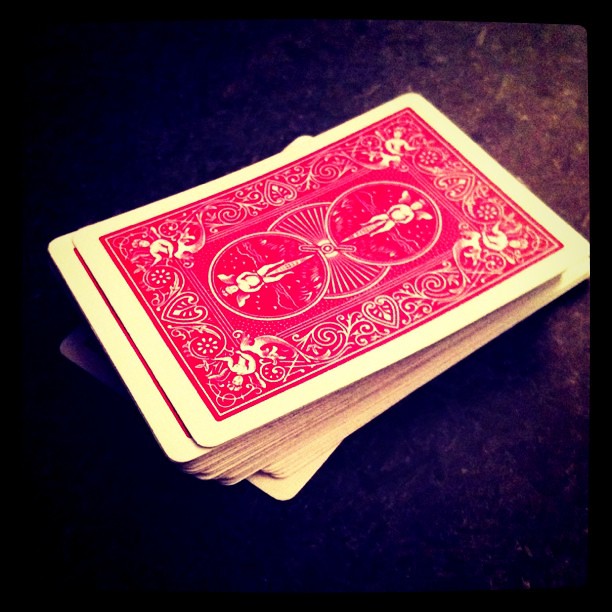A photograph captures a standard deck of playing cards resting on a textured surface, which appears to be either multicolored carpet with predominant brown and maroon tones or dirt. The deck is slightly askew, and you can see the back of one card and a part of the red back of another card. The backs of the cards feature a symmetrical design, common for playing cards, with an illustration of an angel riding a wheel in the center. The red hue of the cards appears slightly unnatural, leaning more towards a rosy shade rather than the usual red typically seen on playing cards. The upper right corner of the image, where the surface texture changes, enhances the rustic ambiance of the scene. The left and right bottom areas of the card are shrouded in shadow, adding depth to the photograph.